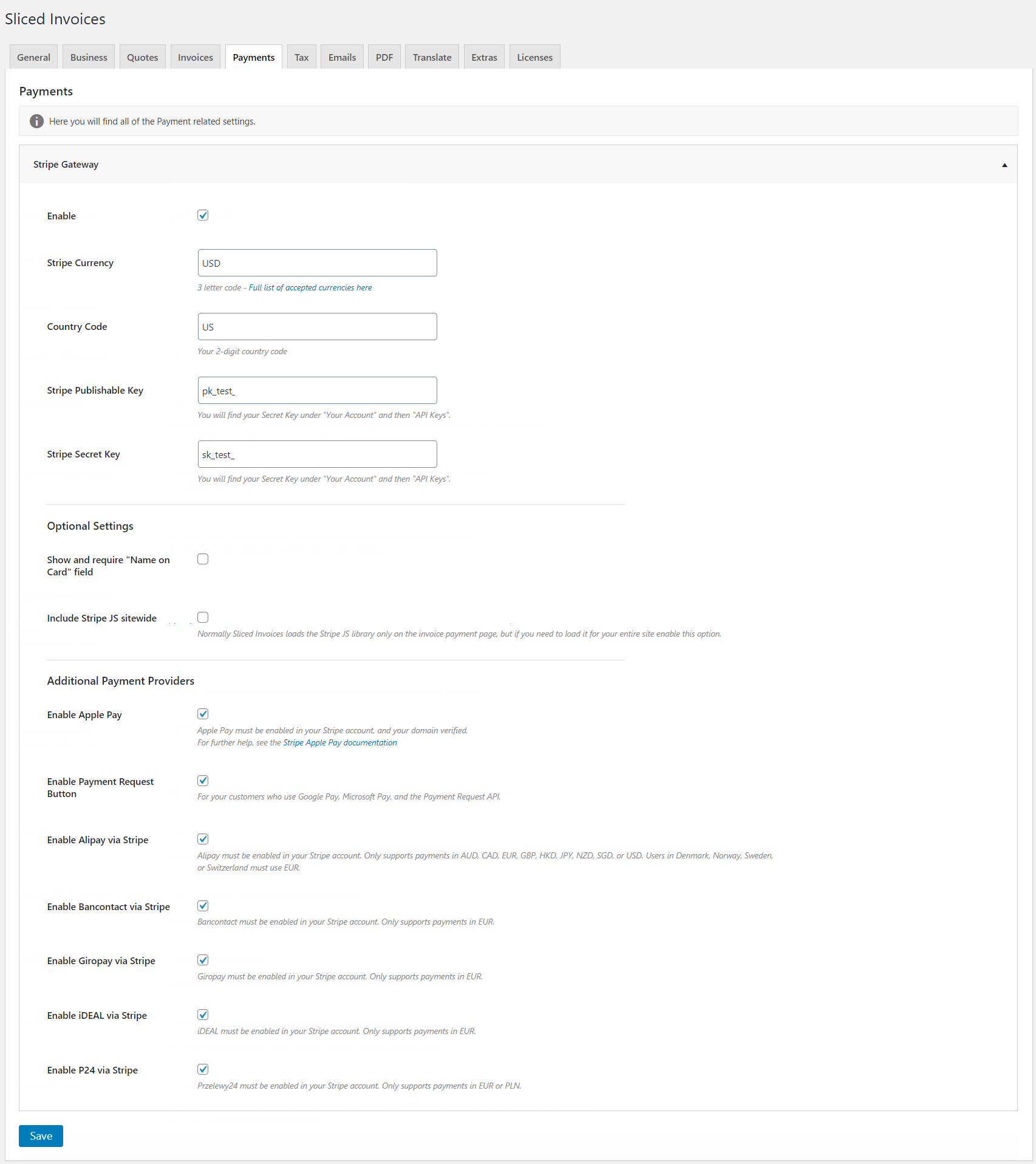The image portrays a vertical interface screenshot, framed against a white background likely illuminated by a computer screen, encompassed by a medium gray border on the sides and bottom. Across the top, a thicker gray rectangular header prominently sits, with the text "Sliced Invoices" in black on the upper left corner. 

Below the header, a series of navigation tabs is visible, including "General," "Business," "Quotes," "Invoices," "Payments" (which is bolded and selected), "Tax," "Emails," "PDF," "Translate," "Extras," and "Licenses." The "Payments" tab features a white background to indicate it is the active selection, while the others have a gray background.

The main content of the screenshot under the "Payments" tab includes a section header stating, "Here you will find all the payment related settings." Below this, there are various settings related to payment configurations. 

Included settings are:
- "Stripe Gateway Enabled" with accompanying options for configurations.
- Fields for "Currency," "Country Code," "Stripe Published Key," and "Stripe Secret Key."
- Additional "Optional Settings" such as requiring a name on the card field and including Stripe 15 site-wide.
- Options for "Additional Payment Providers," with checkboxes next to various enabling settings.

Finally, a prominent blue "Save" button is located at the bottom, intended for saving any changes made to these settings.